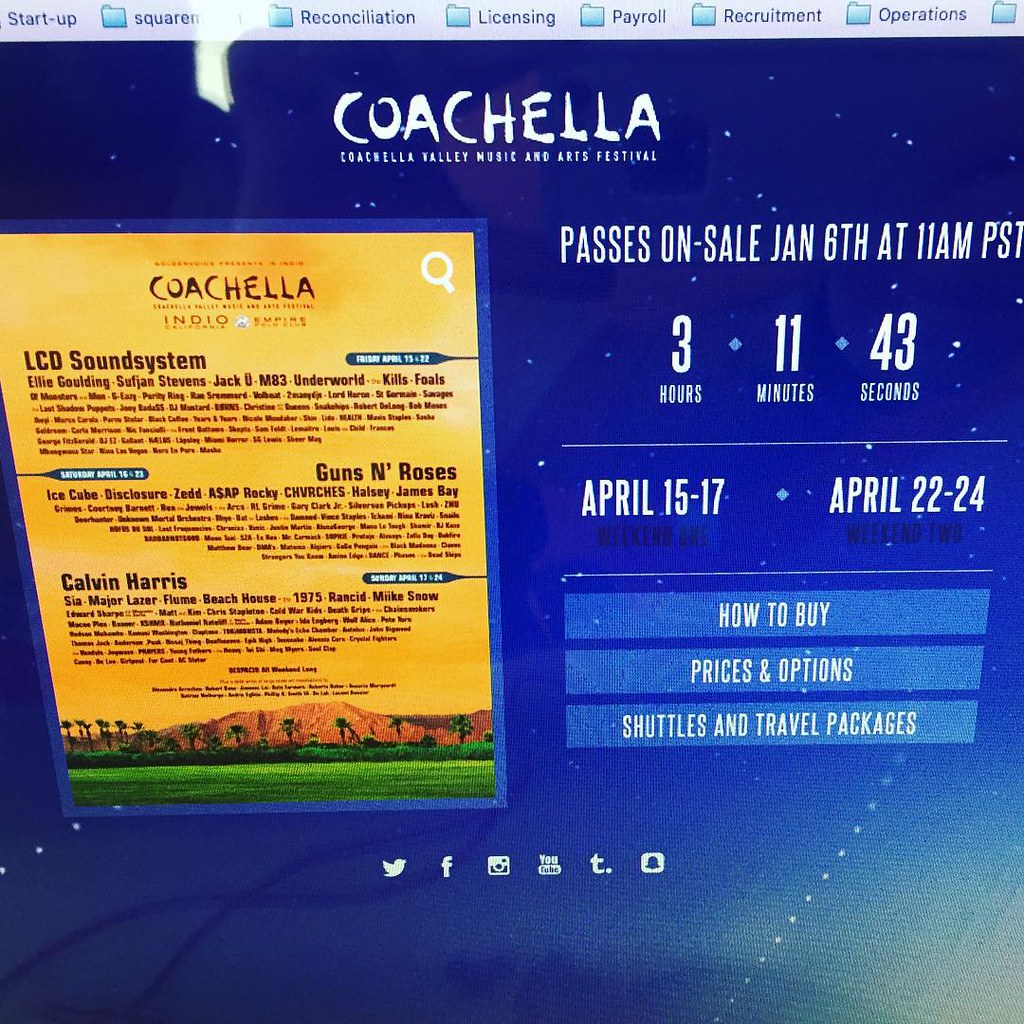This image captures a detailed advertisement for the Coachella Valley Music and Arts Festival displayed on a computer screen. The web browser window showcases folders at the top with labels like Startup, Reconciliation, Licensing, Payroll, Recruitment, and Operations. Dominating the screen is the Coachella advertisement featuring a yellow-hued poster on the left with headlining acts such as Guns N' Roses, Ice Cube, LCD Soundsystem, Ellie Goulding, Calvin Harris, and more. The festival dates are prominently displayed as April 15th-17th and April 22nd-24th, separating the event into two weekends.

In the center-top of the page, white text announces "Coachella, Coachella Valley Music and Arts Festival" and the availability of passes starting January 6th at 11 a.m. PST, accompanied by a live countdown indicating three hours, 11 minutes, and 43 seconds remaining until they go on sale. Below this, three blue buttons provide further information on purchasing options, prices, and shuttle and travel packages. On the bottom left, social media logos including Twitter, Facebook, YouTube, Instagram, Tumblr, and Snapchat are displayed. Overall, the image presents a comprehensive view of the festival's schedule, headliner artists, and purchasing details set against a blue background with white dots.